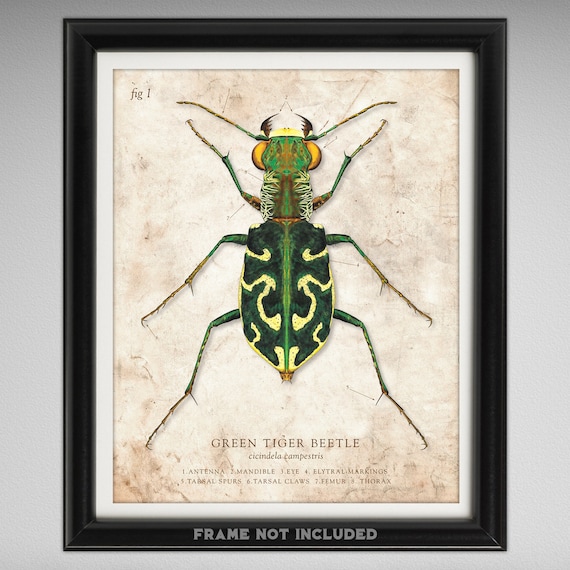The image depicts a large, framed illustration of a "Green Tiger Beetle" hanging on a white wall. The frame itself is black, with the outer background being light gray. The central illustration features a meticulously detailed, top-down view of the beetle, showcasing its vibrant green body adorned with gold wave-like patterns and yellow stripes. The beetle has six legs, arranged three on each side, and two long antennae, each with brown tips. Its head features two prominent orange eyes and distinctive mandibles.

Accompanying the illustration are various labels and annotations. The bottom of the frame includes the title "Green Tiger Beetle," along with a numbered key that identifies different parts of the beetle's anatomy: 1) Antenna, 2) Mandible, 3) Eye, 4) Literal Markings, 5) Spurs, 6) Tarsal Claws, 7) Femur, and 8) Thorax. Additional small text at the bottom of the frame is present but difficult to read. The background of the page holding the beetle illustration is a blend of light gray, white, and hints of light brown.